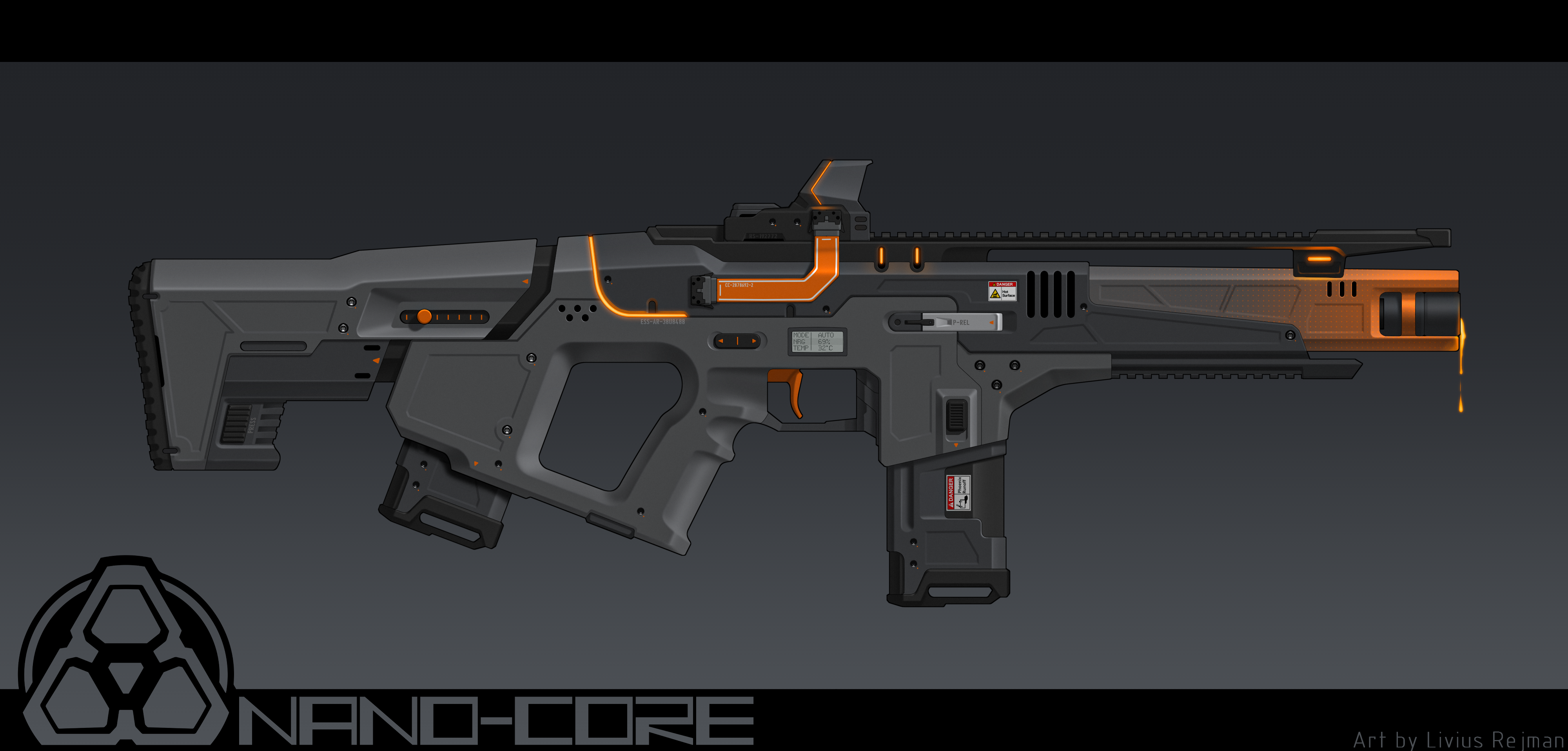This highly detailed rendering depicts a futuristic, stylized rifle designed for a video game. The weapon is predominantly grey with striking orange accents and elaborate detailing, including numerous adjustment knobs, a thick magazine, and a rest for shoulder support. At the top, there is a scope accompanied by small orange highlights. The barrel of the gun is notably oozing a viscous, orange liquid, suggestive of magma or another hot substance, complemented by gradient colors transitioning from orange to light grey. The side of the rifle features intricate details like model numbers, an LCD screen displaying mode settings, and warnings such as "danger, hot surface."

The drawing is set against a dark grey gradient background, which enhances the futuristic and polished aesthetic of the weapon. The bottom of the image features light grey text, with the right corner attributing the artwork to Livis Regman and the left corner displaying the text "Nanocore" alongside a stylistic radioactive triangle logo. The overall composition hints at a speculative design intended for a video game, perhaps depicting a weapon that could offer rapid-fire capabilities given its sleek build and advanced features.